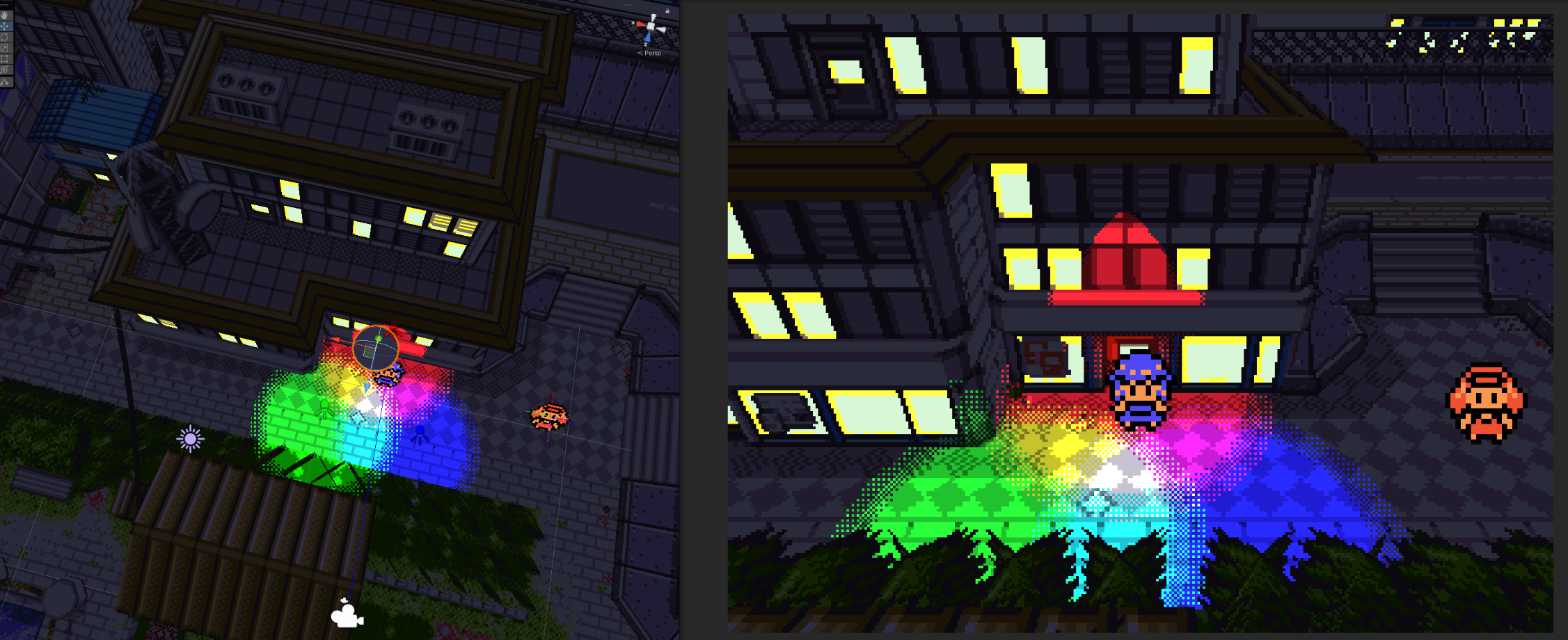The image depicts a pixelated, retro-style computer game from a top-down view and a front view, resembling late 90s indie games. The top-down perspective shows a cityscape with gray stone and concrete buildings, some accented with brown wooden borders and air conditioning units on the roof. The scene includes illuminated windows, green plants, and a shed with a high-pitched brown roof. Various colored spotlights in green, blue, and a yellowish-purple intersect over the area, highlighting the tiled pathways and pixelated trees below. 

The front view provides a close-up of two pixelated characters. One character, wearing a blue outfit, stands on a gray tile where a spotlight shines directly on her. To her right, another character in an orange outfit appears to be emerging from a building. Both have simple black pixelated eyes and minimalistic features. The setup suggests that players must navigate these characters through the city's illuminated paths, interacting with objects and lights to advance in the game. Overall, the image captures the essence of an indie game with its distinct pixelated art style and urban environment.